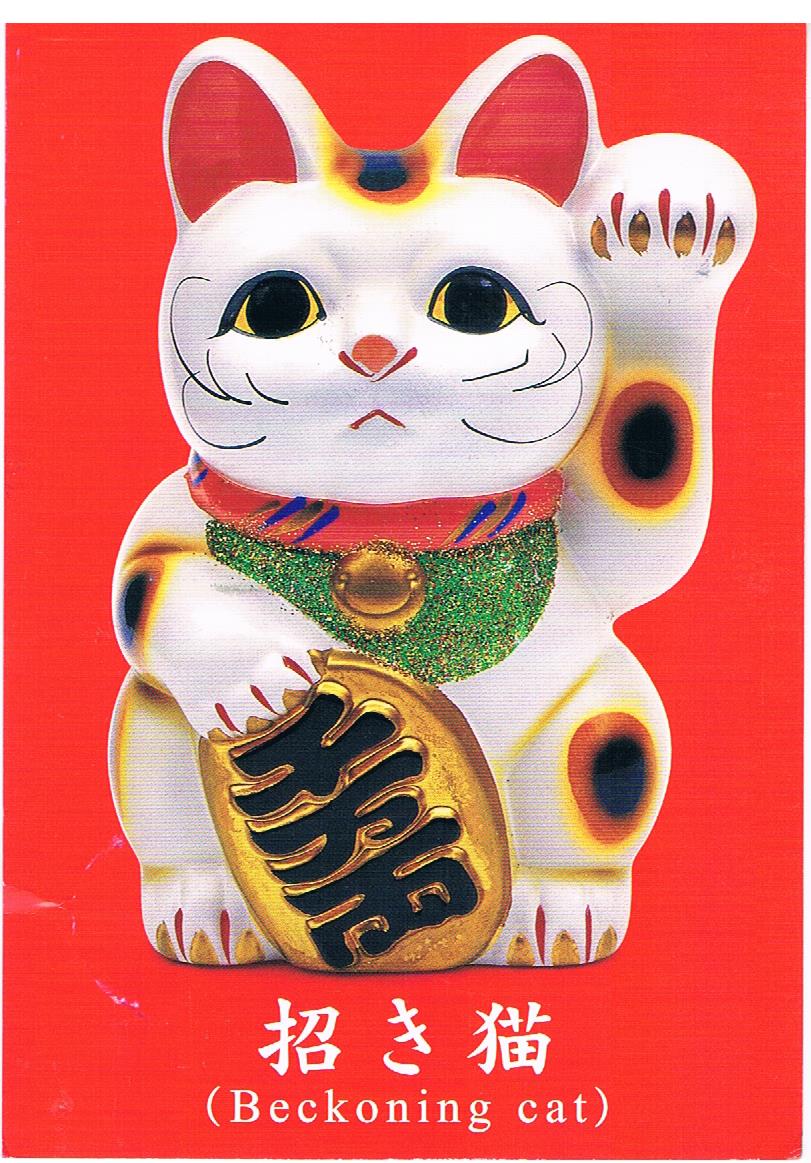The image features a porcelain beckoning cat statue set against a vibrant torch-red background. The cat is predominantly white with intricate details: pink-inside red ears, expressive yellow eyes with black pupils, and a red nose with black whiskers. It sports a red collar adorned with blue stripes and green sparkles, further accentuated by a gold round circle. Notably, the cat's left paw is raised, symbolizing good fortune, while its right paw holds a golden, egg-shaped treasure. The cat's body is decorated with an array of colored spots in black, red, yellow, and orange, including specific detailing on its head, elbows, and knees. Gold-colored claws and red markings delineate the individual fingers. Three white Chinese characters are inscribed at the bottom, translated as "Beckoning Cat".